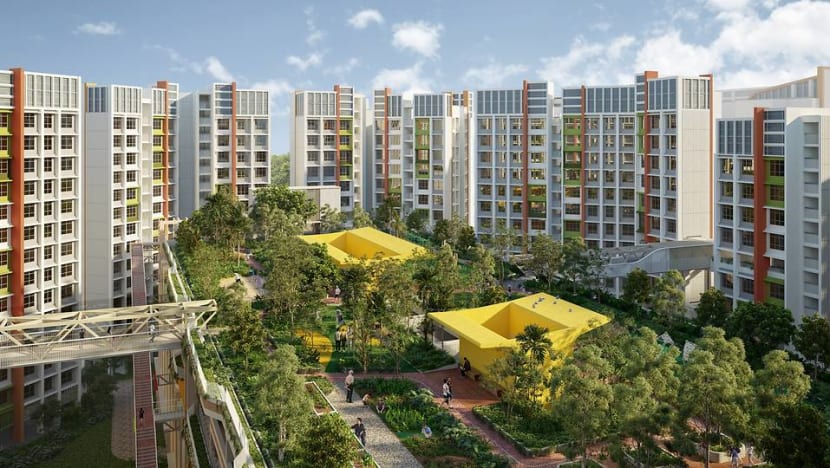This detailed artist's impression depicts the rooftop garden area of a proposed multi-story car park in the Park Residences (PARC) development in Tengah, Singapore. This elevated garden, approximately four to five stories above ground level, is surrounded by numerous apartment buildings, mostly white in color and rising 15 to 20 stories high. The complex is designed to provide low-cost, clean housing and maximize the living space available to its residents.

The rooftop garden features lush greenery with numerous trees, hedges, and beautifully landscaped paths. The walkways, a mixture of red brick and gravel, wind through the space, providing serene walking areas for residents. Seating areas are strategically placed throughout the garden, inviting relaxation amidst the greenery. There are also stairways and bridges that connect different parts of this garden area, including two bridges that extend from the apartment buildings to the garden, further enhancing accessibility.

In the center of the rooftop garden are two distinct yellow buildings with open, cutout roofs. These structures add vibrant color and architectural interest to the overall design. The entire garden is elevated, offering scenic views of the surrounding residential buildings and creating a seamless integration of nature within this urban environment. This thoughtfully designed space not only enhances the aesthetic appeal but also provides a communal area for residents to enjoy, embodying the harmonious blend of urban living and nature typical of Tengah, Singapore.